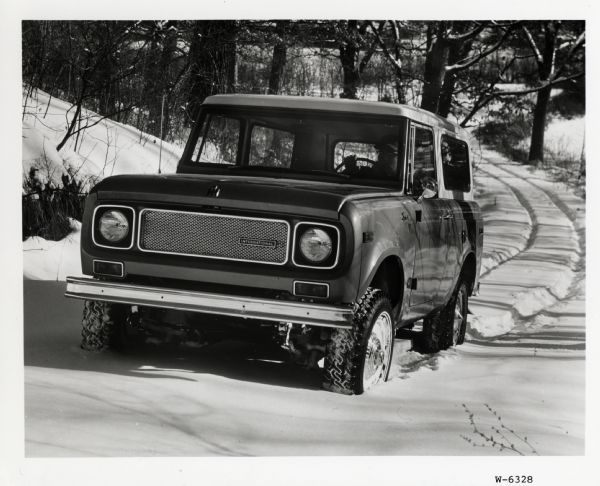This image captures a vintage black-and-white Polaroid photograph of an old SUV driving through a snowy, forested landscape. The SUV is off-center, positioned slightly to the left, and features a visible grille with someone driving, though the driver's details are obscured. The vehicle is traversing an unplowed, snow-covered road, leaving a trail behind it. To the top left, a snowy hill rises, while the top fourth of the background is populated with leafless, dark trees receding into the distance, suggesting a winter setting. The foreground snow shows the tracks made by the SUV's tires as they slush through. A code, "W6328," is marked on the lower right part of the image. The overall aesthetic exudes a vintage feel, likely from the style and composition of the photograph.